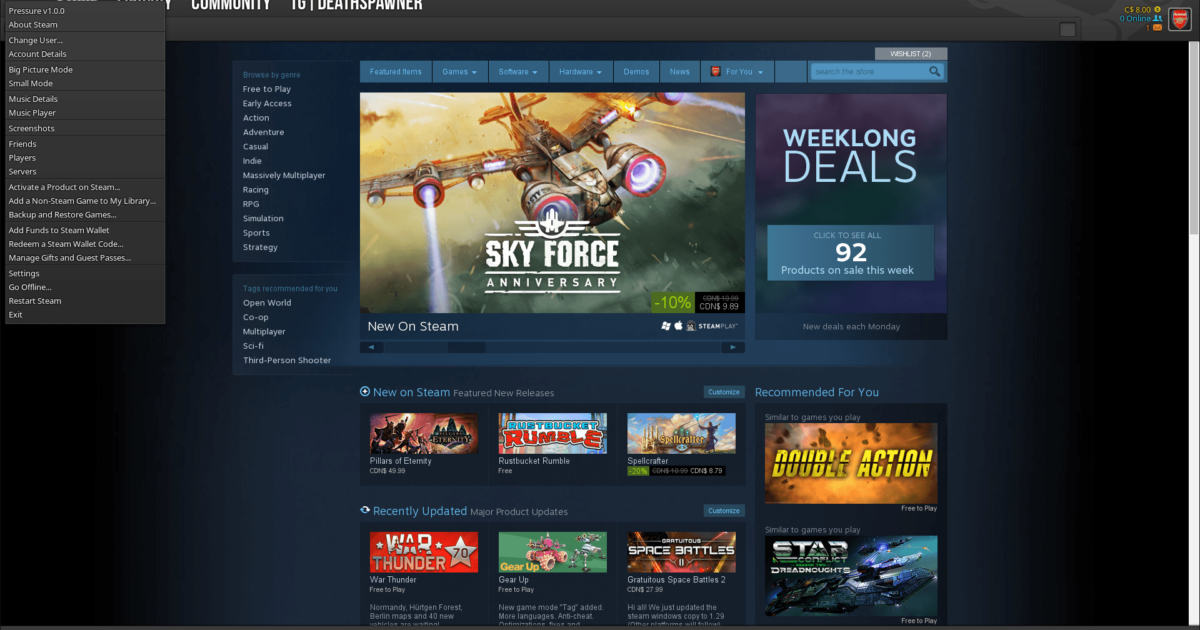The image depicts a webpage from Steam, a popular gaming platform, showcasing a combination of navigation menus and promotional content. On the left side of the screen, there is a tall, vertically-oriented grey menu listing various options such as "Pressure v1.0.0," "About Steam," "Account Details," "Big Picture Mode," "Music Player," "Screenshots," "Friends," "Players," "Servers," "Activate a Product on Steam," "Add a Non-Steam Game to My Library," "Backup and Restore Games," "Add Funds to Steam Wallet," "Redeem a Steam Wallet Code," "Manage Gifts and Guest Passes," "Settings," "Go Offline," "Restart Steam," and "Exit."

In the central part of the webpage, there is a prominent banner featuring the game "Sky Force Anniversary," which appears to be a fighter plane game. Adjacent to this banner is a notification about "Week Long Deals," inviting users to "Click to see all 92 products on sale this week." Below this banner are two rows of three images each, likely showcasing featured games or promotions.

On the right side of the page, there are two larger images under a section titled "Recommended for You," with game titles such as "Double Action," and another game that appears to be "Dragon Dream," following this theme. The cluttered text indicates that the user struggled to interpret the game's names accurately, but it indicates that this section highlights personalized game recommendations.